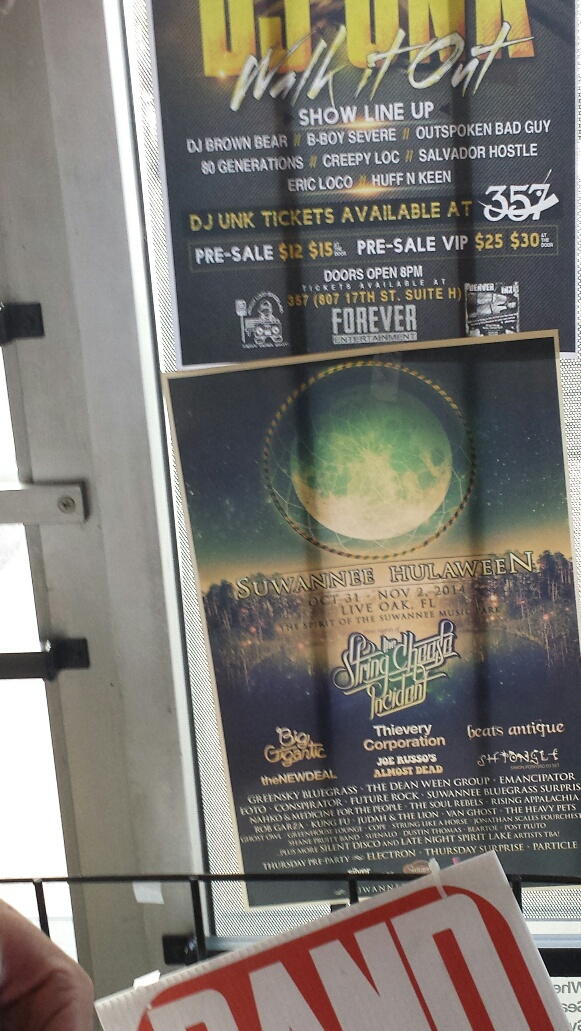The image displays two predominantly black club posters or movie advertisements hanging on a window. The top poster, partially cut off at the top, features yellow text that stands out against a black background. The readable portions include "Walk It Out," "DJ UNK," and "tickets available" followed by the showtimes at 3, 5, and 7. It also lists pre-sale and VIP prices and includes an assortment of emblems along with information on when the doors open. Beneath this, a second poster showcases a moon above a mountain or city structure set against a starry night sky. This poster, featuring green, orange, and black details, mentions "Suwani Hulaween" and "The String Cheese Incident," surrounded by additional information in white and yellow text. The bottom portion of the image reveals a black railing with a red and white sign stating "Banned" and a person's hand barely noticeable in the lower left corner.